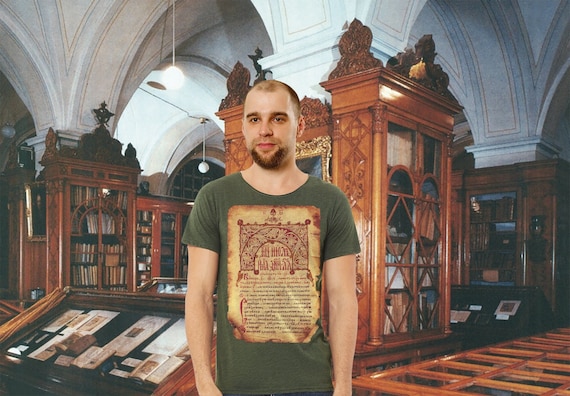Inside a grand Baroque-style building, this photograph showcases the intricate white vaulted ceiling with arches converging in a complex pattern overhead. The room has towering wooden bookcases with glass doors, filled with books, that line the walls and stand prominently in the center. Adding to the library or museum ambiance, the floor is a rich brown wood, and there are ornate glass-topped display cases, one of which is tilted towards the camera, containing various books or placards against a black background. In the immediate foreground stands a young white man with close-cropped receding hair and a reddish goatee, wearing a dark green t-shirt adorned with an illuminated medieval script on the front. The scene captures the essence of a historic setting brimming with literary treasures and architectural elegance.